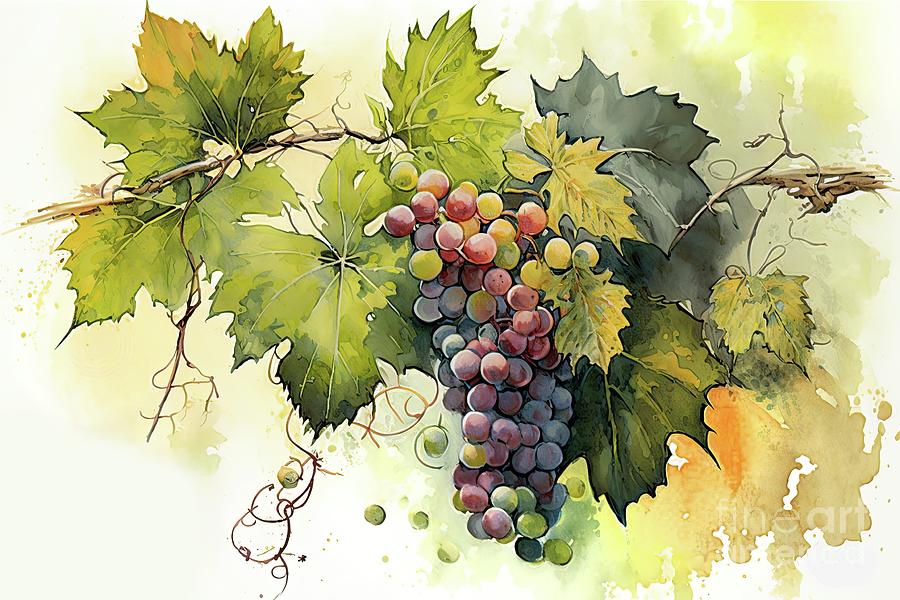This is a beautifully detailed watercolor painting depicting a cluster of grapes on a grapevine. Central to the composition is a bushel of grapes ranging from a dusty yellow-green to deep shades of blue, purple, and purple-gray, giving them a frosted appearance. The grapes are surrounded by large, varied leaves; some leaves exhibit deep green, kelly green, and lime green hues, while others show shades of rust, amber, and even a stark gray. The vine itself appears greenish-gray and winds through the composition, enhancing the focal grapes. The background is abstract, featuring splashes and large spots of pale orange, brown, and green against a white backdrop, emphasizing the watercolor medium. This background also incorporates yellow-green to yellowish-orange tones, lending an artistic, almost ethereal quality to the scene. The painterly textures, as if water has been poured onto the paper, add to the overall charm and delicate intricacy of the artwork.